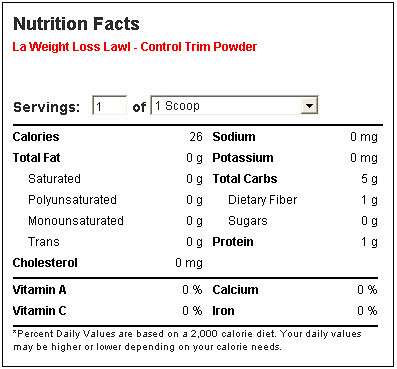This image displays the nutrition facts label of the "LA Weight Loss L-A-W-L-Control Trim Powder" product. The label is presented in black, white, and red colors. Encased in a black border, it prominently features "Nutrition Facts" in black text at the top, followed by the product's name in red. The label details the nutritional content for a single serving size of one scoop, which contains 26 calories. Notably, it contains zero grams of total fat, saturated fat, polyunsaturated fat, monounsaturated fat, trans fat, and zero milligrams of cholesterol, sodium, and potassium. The total carbohydrates amount to 5 grams, including 1 gram of dietary fiber and zero grams of sugar. The protein content is listed as 1 gram. Additionally, vitamins and minerals such as Vitamin A, Calcium, Vitamin C, and Iron are all indicated at zero percent daily value. At the bottom, a disclaimer notes that the percent daily values are based on a 2,000 calorie diet and may vary depending on individual calorie needs. The label itself is straightforward, set against a white background, with the information organized clearly in a box layout.